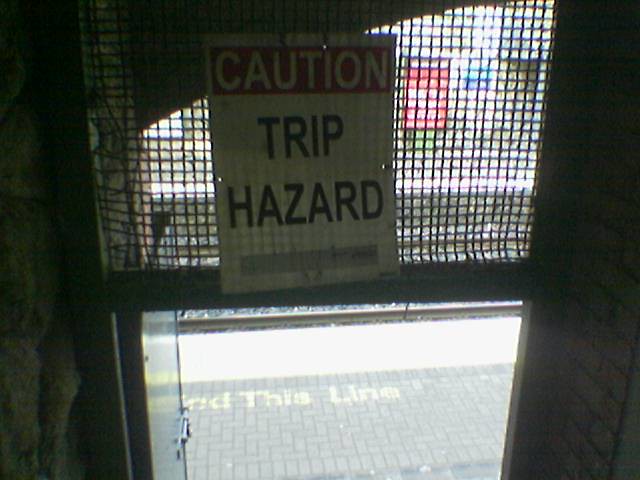The image depicts the inside view of the top portion of a door within a building, where a metal fence structure made up of small square grids spans across the top. Hanging on this metal fence is a white sign featuring a red bar at the top with the word "CAUTION" in white letters, and below it, the words "TRIP HAZARD" in black. Beneath this setup, on the left side, a grey metal door stands open, leading to the outside. The exterior appears to be a street paved with grey bricks, where yellow-painted text reading "THIS LINE" is visible on the ground.